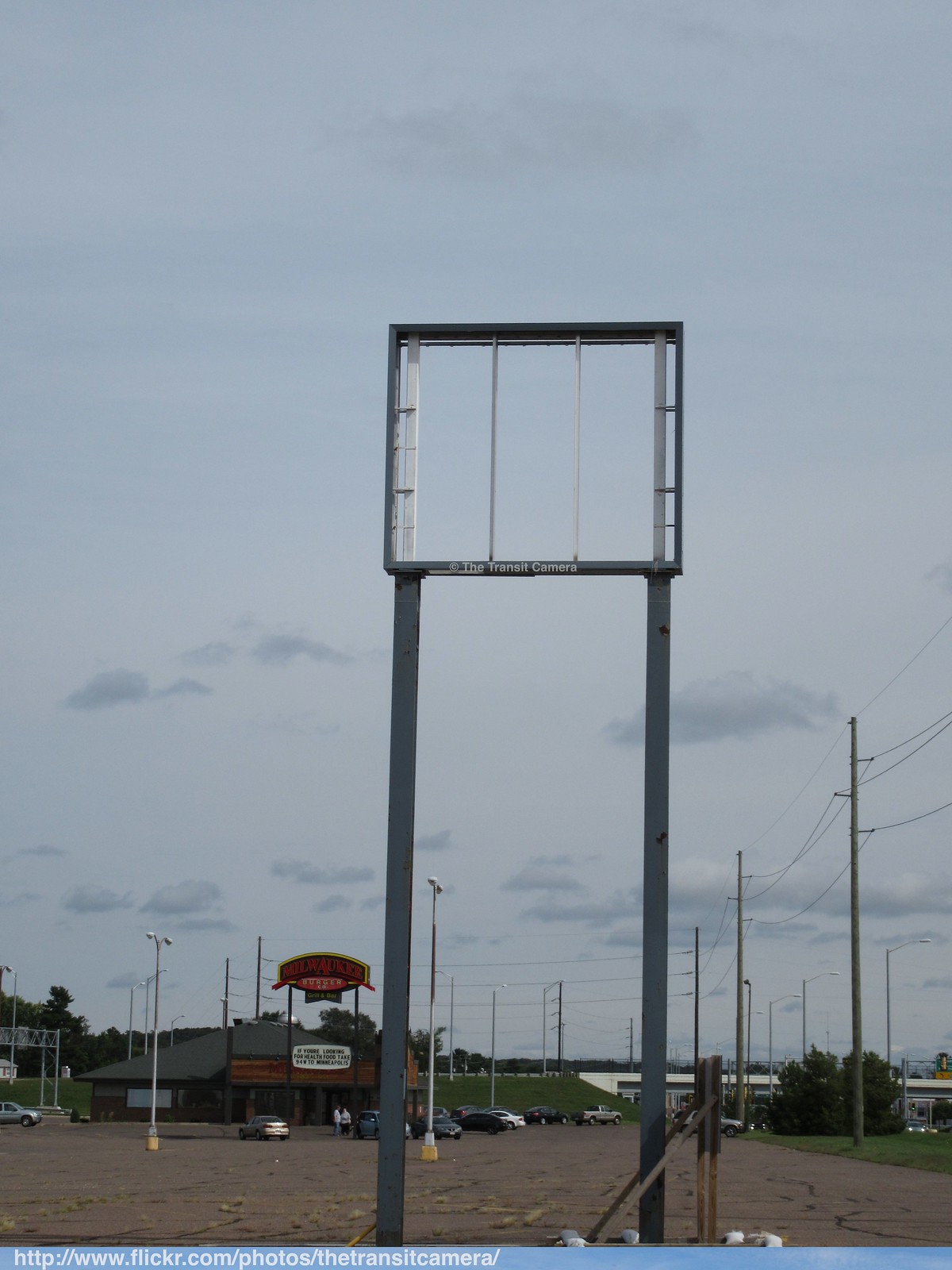A photograph depicts an unused parking lot, evident from grass sprouting through the pavement, beneath a cloud-filled, bluish-gray sky. Dominating the scene are two gray-colored metal posts with white brackets forming a square frame meant for a sign, though currently empty. The structure bears a copyright notice reading "The Transit Camera." In the distance, a red and yellow marquee for the "Milwaukee Burger Company" restaurant is visible, surrounded by a parking lot with several cars. Beyond the restaurant, a grassy hill rises, completing the backdrop. In the bottom left corner of the image is the text "http://www.flickr.com/photos/thetransitcamera."